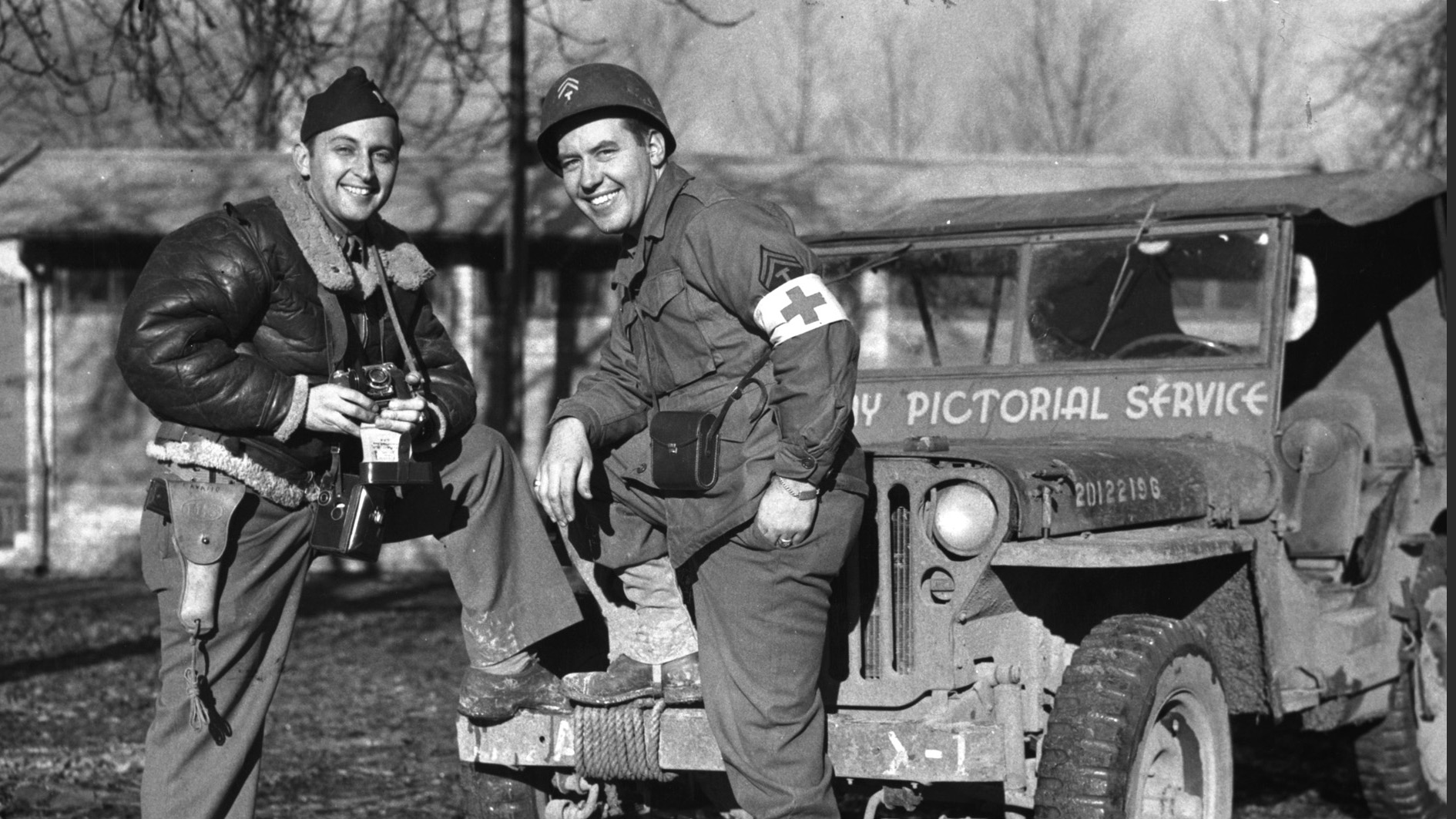This black-and-white photograph captures a moment during World War II, depicting two soldiers outdoors amidst a winter landscape, evidenced by the barren tree branches and overcast sky. Dominating the scene is a one-story wooden building, probably a barracks, and a small military jeep without doors but with a raised canvas convertible top. The jeep, positioned to the right, bears the designation "Pictorial Service" across its front and a serial number "201-22196" along the side of the hood.

In the foreground, two Caucasian soldiers stand with one leg resting on the jeep’s front bumper. They are engaged with each other yet looking directly at the camera, conveying a sense of camaraderie and purpose. The soldier on the left is dressed in a heavy dark leather jacket with fur trim, military pants, and a cap. He is heavily equipped with several cameras around his neck and a holstered pistol at his side, smiling confidently.

The soldier to the right is identified by a white armband with a cross, indicating his role as a medic. He sports a dark gray button-down jacket, military uniform, and a domed helmet adorned with insignia, suggesting a technical rank. A camera hangs from his shoulder, resting casually at his hip, adding to the narrative of documentation and support during the war.

The overall atmosphere of the image evokes a mixture of melancholy due to the winter setting and a sense of duty and determination reflected in the soldiers' expressions and postures.